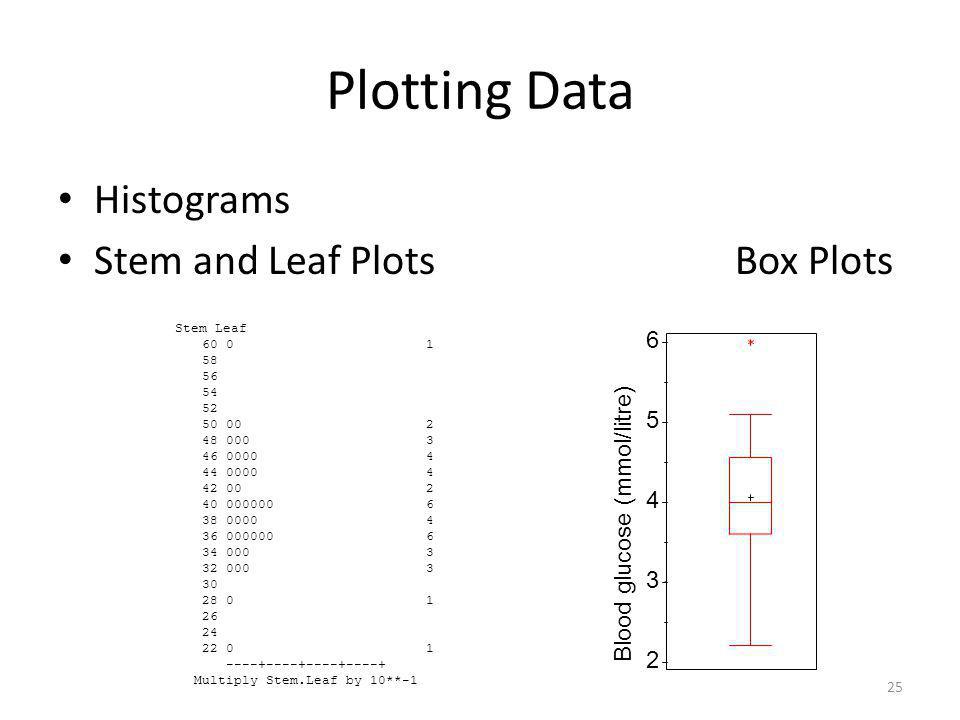The image is titled "Plotting Data" prominently in the center. On the left side, there are two lines of text: "Histograms" and "Stem and Leaf Plots," positioned above a graph. The x-axis of the graph reads "multiply stem.leaf by 10 times times minus 1," and the y-axis ranges from 22 to 60, labeled "stem.leaf." Additionally, zeros are shown near the left side of the graph, while the right side displays numbers in sequence: 1, 2, 3, 4, 4, 2, 6, 4, 6, 3, 3, 1, 1, with 1 at the bottom. 

To the right is another section labeled "Box Plots" above a long rectangular graph measuring blood glucose levels in mmol/L. This graph features two short red lines; one slightly above 2 and another slightly above 5 on the y-axis. Vertical lines extend from the top and bottom horizontal lines, converging at a rectangle in the graph's center. Inside the rectangle, a horizontal line is positioned near the middle, aligning with the number 4 on the y-axis.